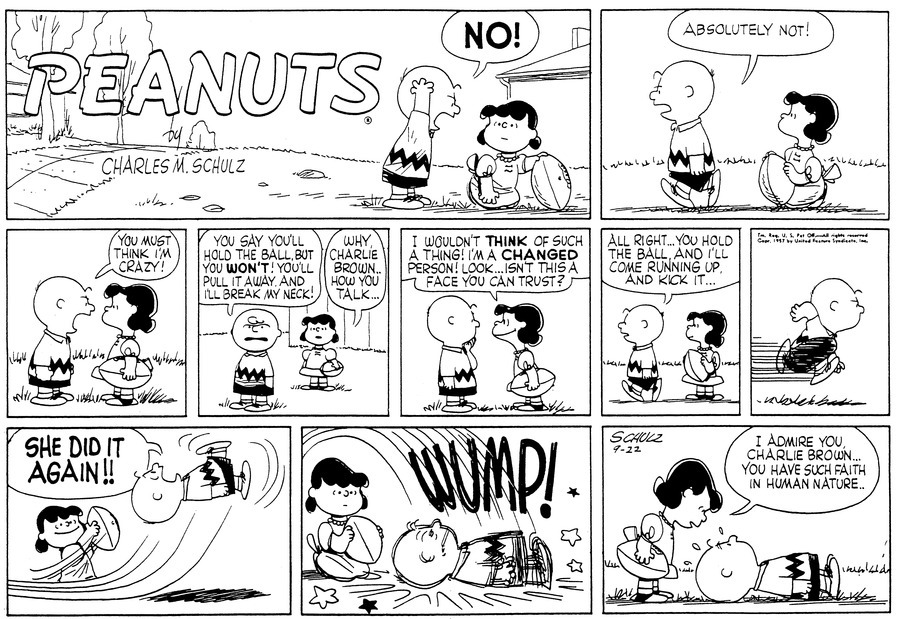This black-and-white comic strip from "Peanuts" by Charles M. Schulz features a humorous interaction between Charlie Brown and a girl holding a football. The comic begins in the top left corner with the iconic title "Peanuts by Charles M. Schulz." The strip is divided into three segments: the first segment has two scenes, the second has five, and the third has three. In the initial scene, Charlie Brown, the small boy with a round head, stands on a front lawn and screams "NO!" at the girl who is holding a football. He then exclaims "Absolutely not!" as he walks away from her. Despite his reluctance, the girl convinces him to try kicking the football. The comic culminates in a classic comedic moment where, just as Charlie Brown goes to kick the ball, she pulls it away, causing him to fall flat on his back with a "Wump!" sound effect. The final scene shows the girl standing over a supine Charlie Brown, saying, "I admire you, Charlie Brown. You have such faith in human nature." In the top left corner of the last panel, Schultz's signature "Schultz 922" is visible, marking his authorship and the date.